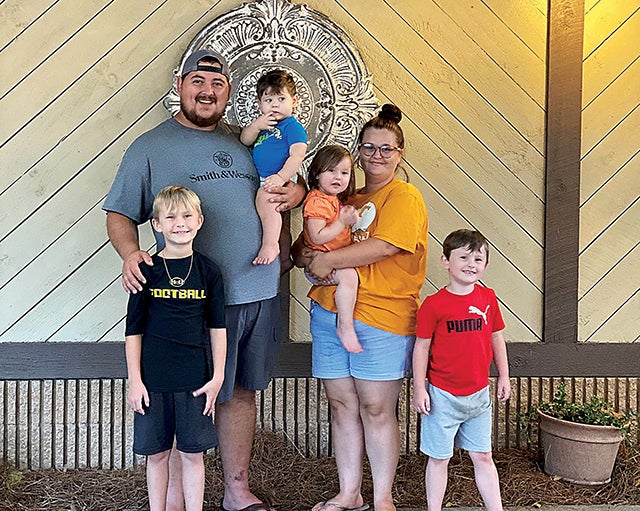In the photo, a cheerful family of six stands together against a decorative wall made of light and dark wooden planks. On the lower right-hand corner, a potted plant adds a touch of greenery to the scene. The ground beneath them is covered in hay, suggesting an outdoor setting. The father, standing on the left, is a heavyset man wearing a gray T-shirt with "Smith and Walensky," possibly a reference to the seafood restaurant, short pants, sandals, and a backward gray baseball cap. He holds a chubby baby boy dressed in a bright blue T-shirt, who has his right finger in his mouth. The father's right hand rests on the shoulder of his eldest child, a seven or eight-year-old boy with blonde hair, who is dressed in a black T-shirt with the word "football" and black shorts, and wears a necklace.

The mother, to the right of the father, is slightly shorter by about six or seven inches, standing approximately 5'4" to 5'5". She is a bit overweight and wears glasses along with her hair in a bun. Her outfit consists of a bright orange T-shirt, blue jeans, and flip-flops. She is holding a young daughter who appears to be around two and a half to three years old, wearing an orange T-shirt. Next to the mother is another son, about five years old, with black hair and a cute smile. This child is dressed in a very bright red Puma T-shirt and light-colored blue jeans. All family members are sporting colorful T-shirts paired with more muted shorts or pants, fitting the casual and relaxed nature of their ensemble.